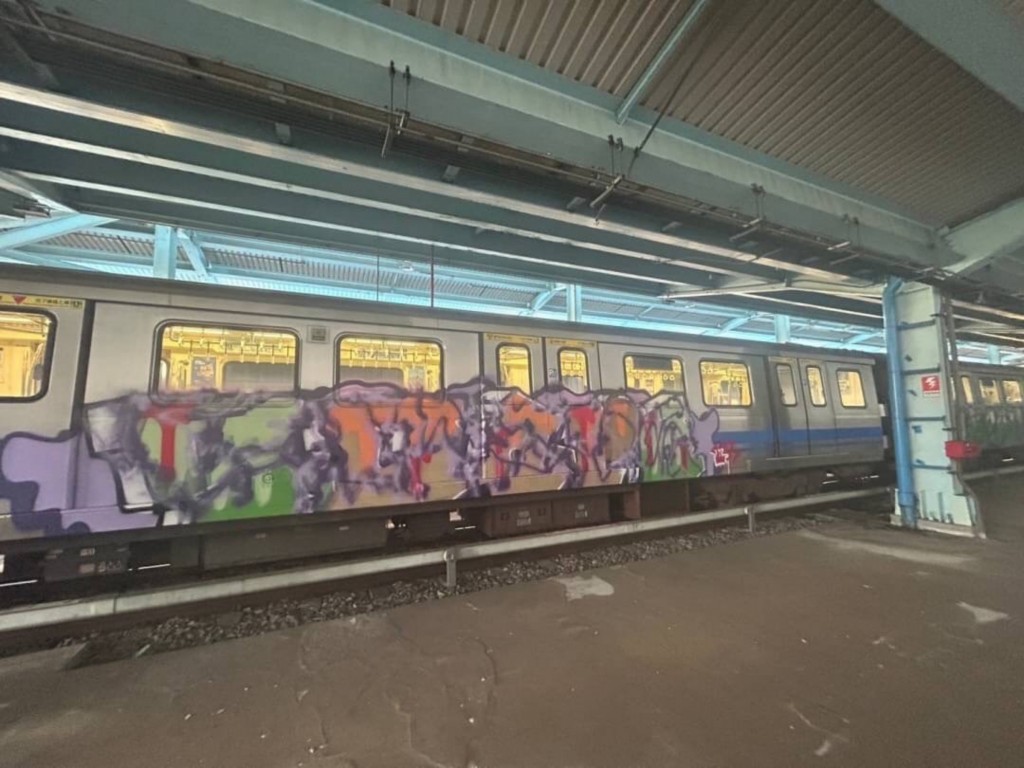This image captures a deserted subterranean subway station. Dominating the scene is a long subway car, extending the full width of the picture. The exterior of the subway car is heavily covered in multicolored graffiti, with prominent hues including orange, red, and green. Despite the apparent effort, the graffiti forms an indistinguishable amalgamation of shapes and letters.

Above the subway car runs a ceiling with an industrial, textured metal finish, equipped with support beams and silver pillars. The ceiling also carries blue and aquamarine lighting that illuminates the scene with an overlay of cool tones. Inside the subway car, the lights are on, casting a soft yellow glow through the windows, yet no passengers are visible either on the train or the platform. This, coupled with the complete absence of people on the cement platform floor, suggests that it may be late at night or that the car is out of service. Various structural details are visible, including rails, support pillars, and directional signage indicating loading and exit doors. The overall lighting creates a stark, almost eerie atmosphere in the otherwise vividly painted setting.